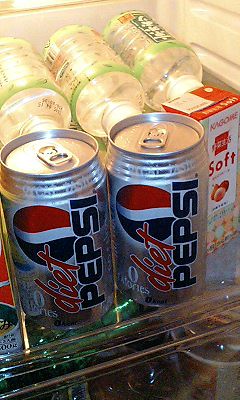This image provides a detailed look inside a refrigerator, focusing on a clear glass or plastic shelf and a partial view of the drawer beneath it. Prominently displayed on the shelf in the foreground are two silver cans of Diet Pepsi, each adorned with a circular logo featuring a red top, a swishy white stripe, and a blue bottom. Just behind the cans, there are three bottles of water arranged in a vertical stack, with another layer of three bottles visible underneath. The water bottles are clear and sport a green and clear label. An orange and white box labeled "Soft" is situated behind these stacks. The refrigerator's back wall is white with horizontal indented stripes. Below the glass shelf, the edge of another drawer is visible, containing assorted items. In the left corner of the image, there's a glimpse of another box with an orange and white label, distinct from the first box.